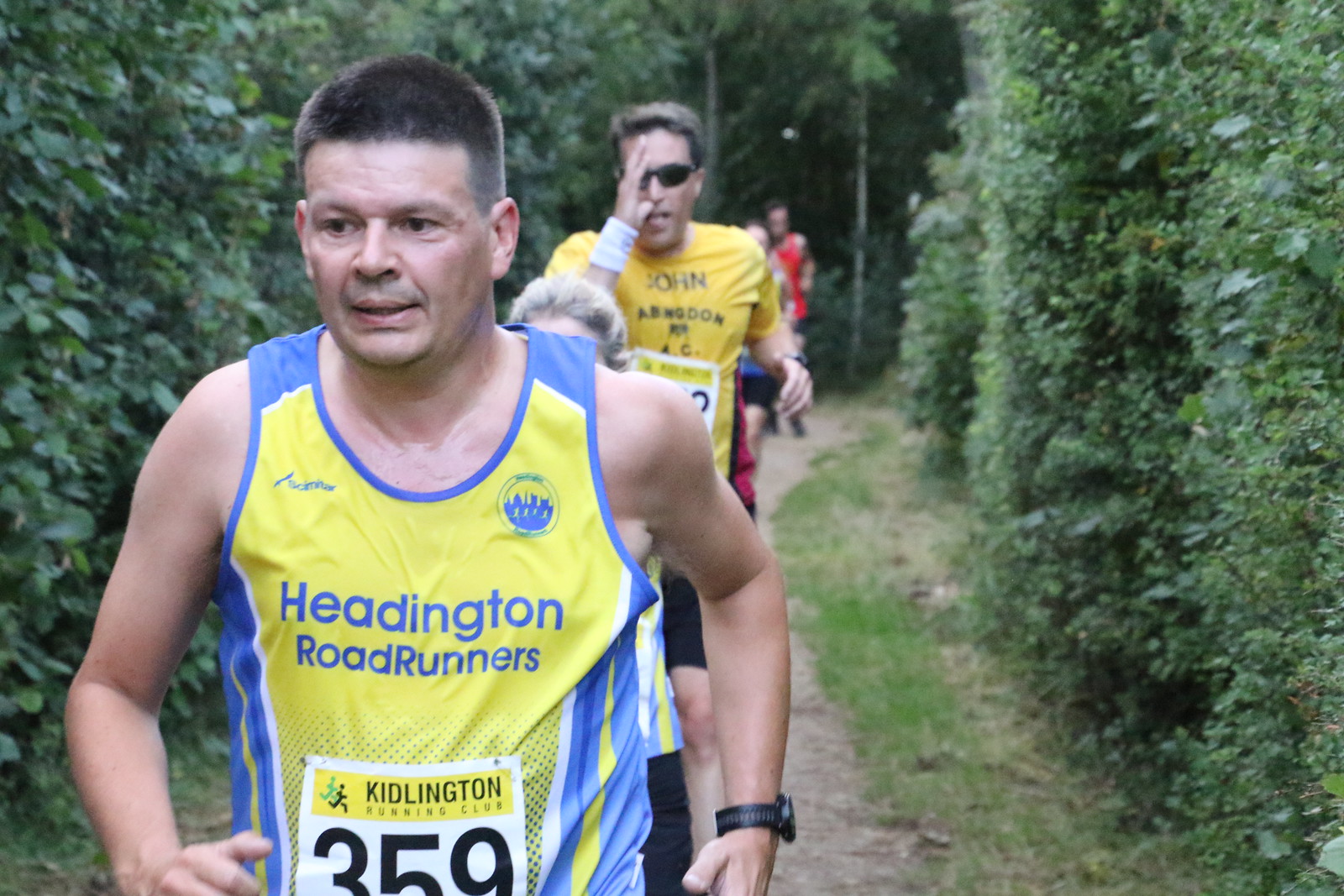This photograph captures a vibrant moment in a cross-country running race taking place on a narrow, dirt trail winding through a lush, green forest. The trail is lined with manicured hedges and dense greenery on either side. Leading the line of runners is a middle-aged Caucasian man with short, buzzed brown hair, wearing a blue and yellow tank top that reads "Headington Road Runners." Affixed to his abdomen is a white race bib labeled "Kidlington Running Club" with the number 359.

Directly behind him is an older woman with short gray hair, partially visible, who is also wearing a blue and yellow jersey. The third runner in line is a tall gentleman in sunglasses, clad in a yellow t-shirt that reads "John Abingdon" on the front. He has a white wristband on his right wrist and his left arm is bent at the elbow as he runs. The line stretches back into the forest, with the furthermost runner discernible only by a bright red top, fading into the greenery. The photo vividly captures the serene yet focused atmosphere of the marathon, though the exact location is unspecified.